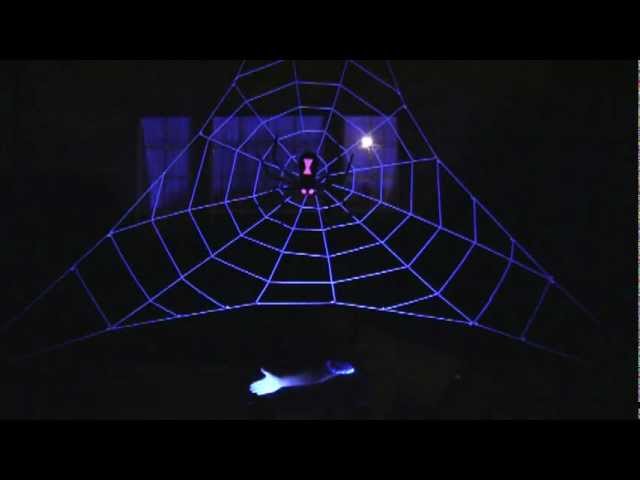This is a highly detailed digital image featuring a dramatic and eerie scene. Set against an entirely black background, the focal point of the image is a large, triangular-shaped spider web radiating from the center, illuminated by a captivating bluish-purple light. At the center of the web, a menacing black widow spider is perched, distinguished by its iconic red hourglass marking and strikingly glowing red eyes. The backdrop of the web showcases a purplish bay window with three distinct segments, through which shines the full moon, casting a surreal light over the scene. Below the spider web, there is an iridescent, glowing human arm, disjointed just below the shoulder, lying eerily with the thumb splayed outwards. The combination of the glowing spider, the ethereal light from the bay window, and the disembodied, glowing arm contributes to a hauntingly surreal atmosphere.